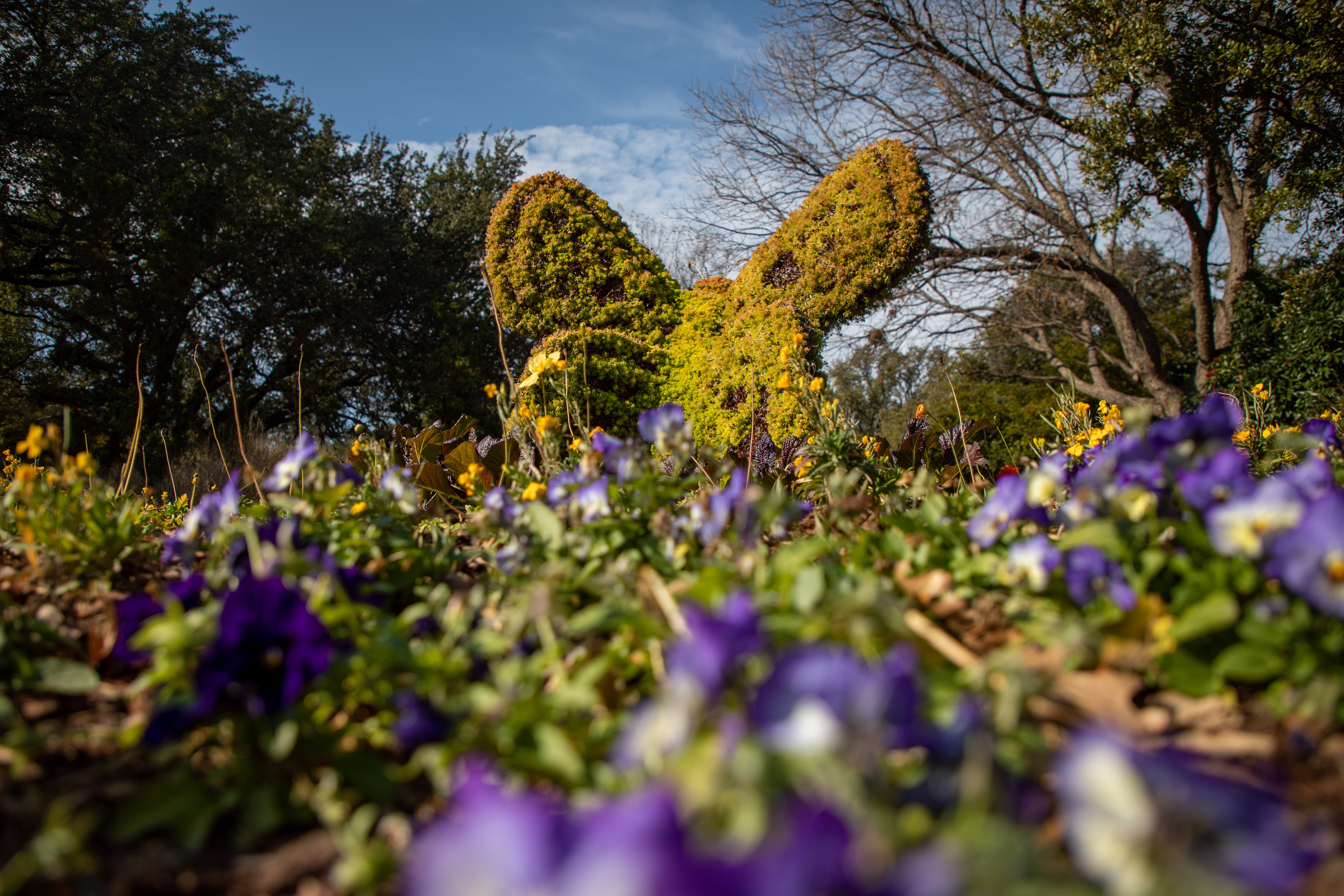This image captures a vibrant garden scene from a low angle, giving a detailed perspective of the lush greenery and colorful flowers below. In the foreground, an abundance of green leaves and vibrant, purplish-violet flowers with yellow centers dominate the view, some slightly blurred to enhance the depth. As your eyes move towards the center, you see a meticulously trimmed topiary, potentially a bush or moss-covered sculpture. This topiary is creatively shaped, resembling a bunny with its two large ears standing upright, although some might interpret it as having wings like a butterfly or even as an unusual cactus form. The backdrop consists of numerous trees on both sides, framing the garden scene. Above, the sky is a serene dark blue with wispy white clouds, indicating a sunny day. The overall composition combines the detailed flora in the foreground with the artistic and whimsical green sculpture, creating a picturesque and enchanting outdoor space.